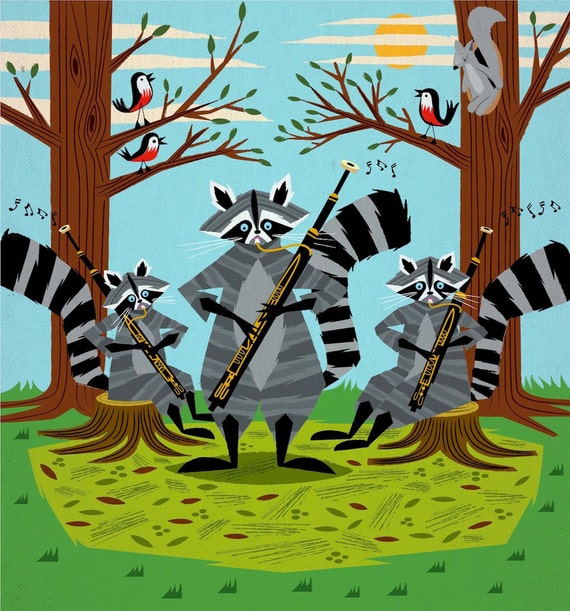In this detailed illustration, three raccoons, predominantly grey with bushy, black-striped tails, are captured engaging in a musical performance. The central raccoon is standing while playing a black bassoon adorned with golden trimmings, creating a focal point in the artwork. Flanking this raccoon are two others, each sitting on a tree stump, also playing similarly detailed bassoons. Behind them, two tall trees with brown trunks and verdant leaves rise, featuring birds perched on branches—two on the left tree and one on the right. These birds, with vibrant red, white, and black plumage, appear to be tweeting or singing, adding to the musical ambiance.

To the right, a grey squirrel is seen sitting within a hollow of the tree, intently listening to the raccoon trio’s performance. Musical notes emanate from the bassoons, suggesting a lively tune fills the air. The ground is a lush green carpet of grass with scattered leaves, under a sky painted in shades of blue accented by wispy white clouds and a glowing yellow sun. This charming scene embodies a whimsical style, where animals take center stage in a harmonious symphony against a vibrant, natural backdrop.